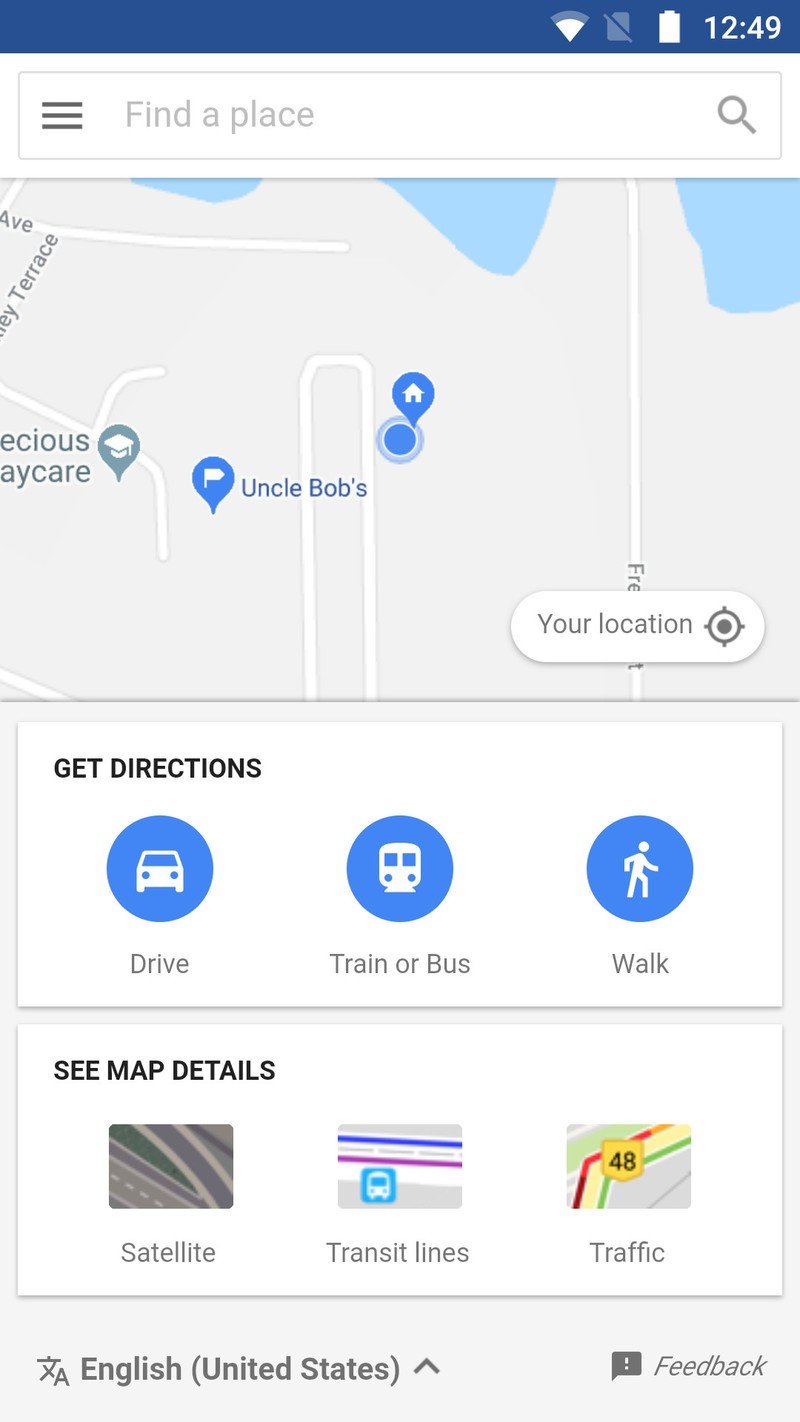At the top of the image, there is a long rectangular bar colored dark blue. Inside this bar, a white battery icon is positioned vertically, indicating a full charge. Beside the battery icon, the time is displayed as 12:49. Beneath the bar, there is a search field with three small horizontal lines on the left, and the light gray text "Find a place" within it. To the right of this text, there is a search icon.

Below the search bar, a map area is displayed with a light gray background. On the map, there are several blue circles, likely representing bodies of water. Key locations are marked on the map: "Uncle Bob's" is noted next to a blue circle, "Precious Daycare" is located further left, and there is a dark green circle containing a graduation cap emblem.

In the bottom right section of the map, the text "Your Location" appears with the phrase "Get Directions" in black underneath it. Below this, three blue circular icons indicate different modes of transportation: a white car for driving, a vehicle for train or bus transport, and a person icon for walking.

Further down, the text "See Map Details" provides additional options such as "Satellite," "Transit Lines," and "Traffic." These options are accompanied by a square containing yellow, red, and green lines, symbolizing traffic conditions, with the number 48 in the center.